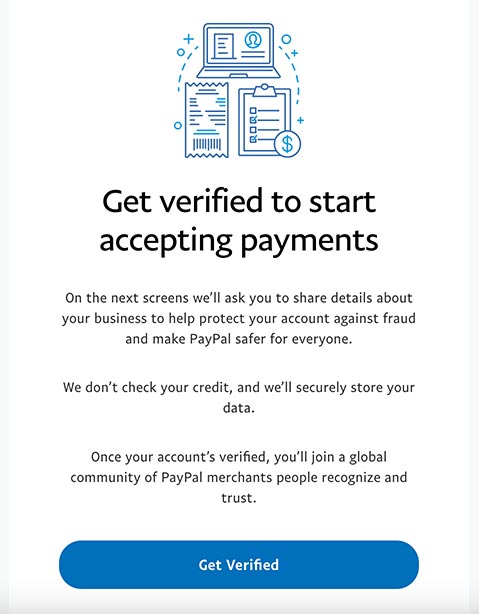This is a portrait-oriented screenshot of a PayPal verification screen, set against a white background. The image is bordered in gray on the left, right, and bottom edges, with no border at the top. Dominating the top-center of the screenshot is an outline illustration of an open laptop, from which dashed lines extend downward in a circular pattern. These lines connect to an outline drawing of a clipboard on the right and a receipt on the left, interspersed with several 'O' shapes and plus symbols.

Directly below this graphic, bold text prompts users with the message: "Get verified to start accepting payments." It is followed by additional text explaining the process: "On the next screens, we'll ask you to share details about your business to help protect your account against fraud and make PayPal safer for everyone. We don't check your credit and will securely store your data. Once your account is verified, you'll join a global community of PayPal merchants people recognize and trust."

At the bottom of the screenshot, a wide blue button features centered white text reading "Get Verified," inviting users to initiate the verification process.